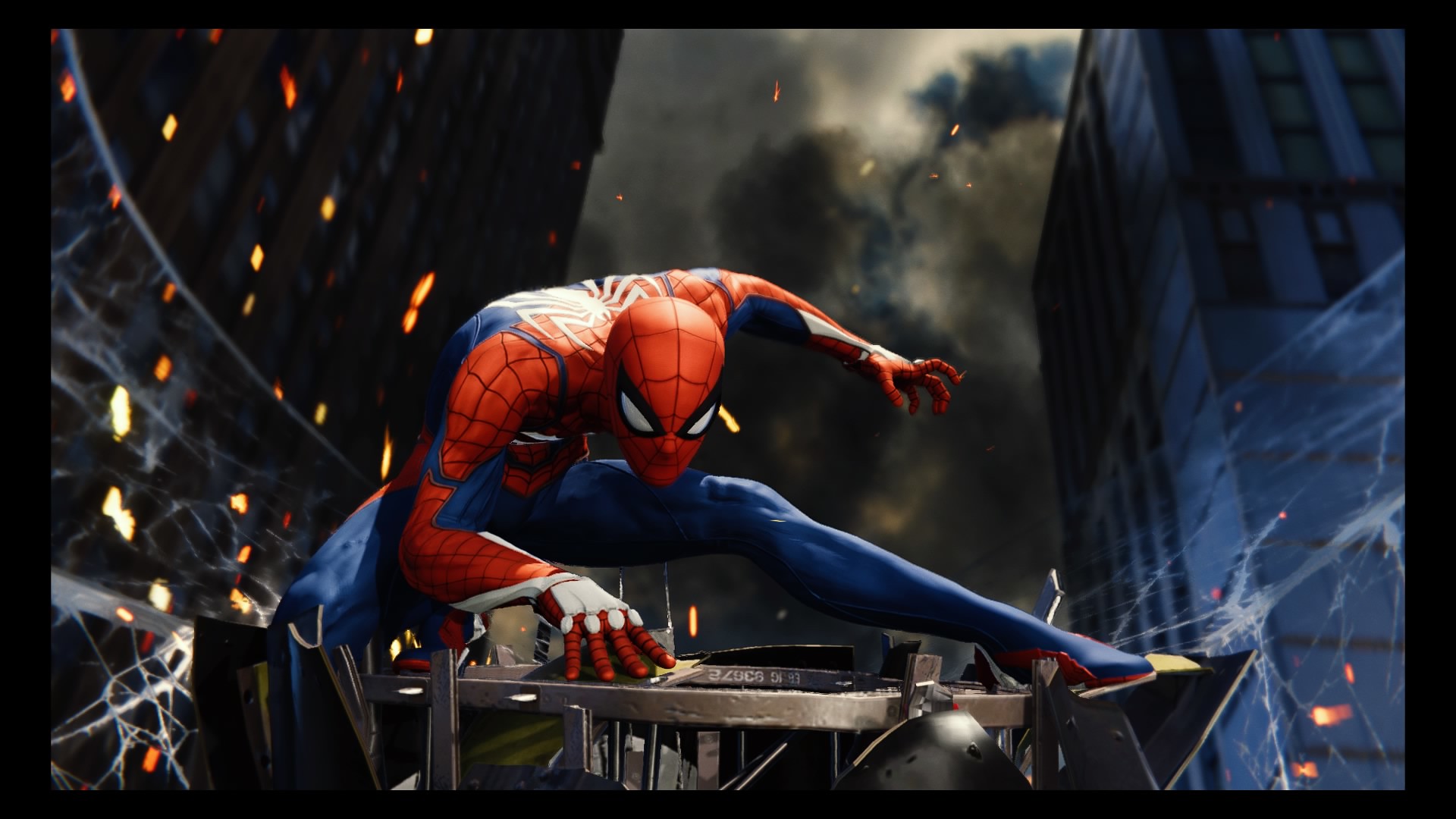This high-tech, action-packed image, likely sourced from a video game or animated series, features Spider-Man in a dramatic nighttime cityscape. Dominating the scene, Spider-Man crouches on a metal structure amidst tall buildings, his iconic red and blue suit adorned with a detailed web pattern and the distinctive spider emblem on his chest. His dynamic posture is full of tension and readiness—his left leg stretched out and his right leg bent behind him, with his right hand gripping a metal object and his left arm extended, poised to shoot webs. The surrounding environment heightens the tension, with smoke and debris floating in the air, illuminated by the fiery glow of an explosion in the background. The sky is gloomy, filled with dark gray and white clouds, creating a dramatic backdrop against the silhouetted, light-speckled buildings. The intricate lighting adds to Spider-Man's resolute gaze directed towards the camera, accentuating the high stakes of what appears to be an intense battle or rescue mission.